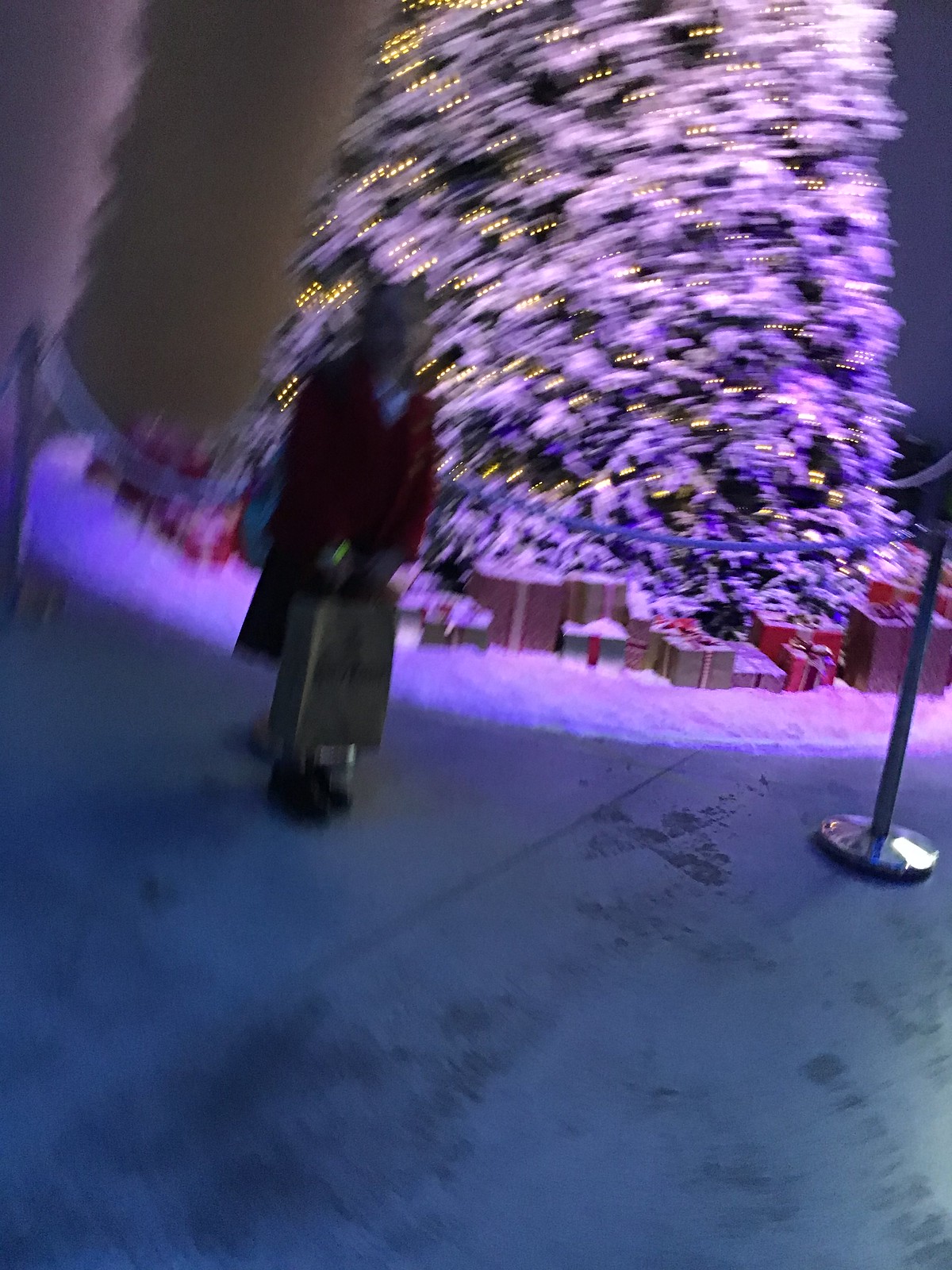This extremely blurry color photograph captures a festive scene set on a dark gray floor. Dominating the background is a large Christmas tree dusted with what appears to be artificial snow, and adorned with numerous twinkling white lights that create a soft, glowing blur. Around the tree's base, a ring of artificial snow encloses a variety of wrapped presents, hinting at holiday cheer. The tree is cordoned off by a blue security rope connected to a metal post situated at the right side of the image, adding a subtle hint of order to the festive display. Standing slightly off-center to the left is a person, whose red coat and brown shopping bag are discernible despite the photograph's blurriness, adding a human element to the scene.